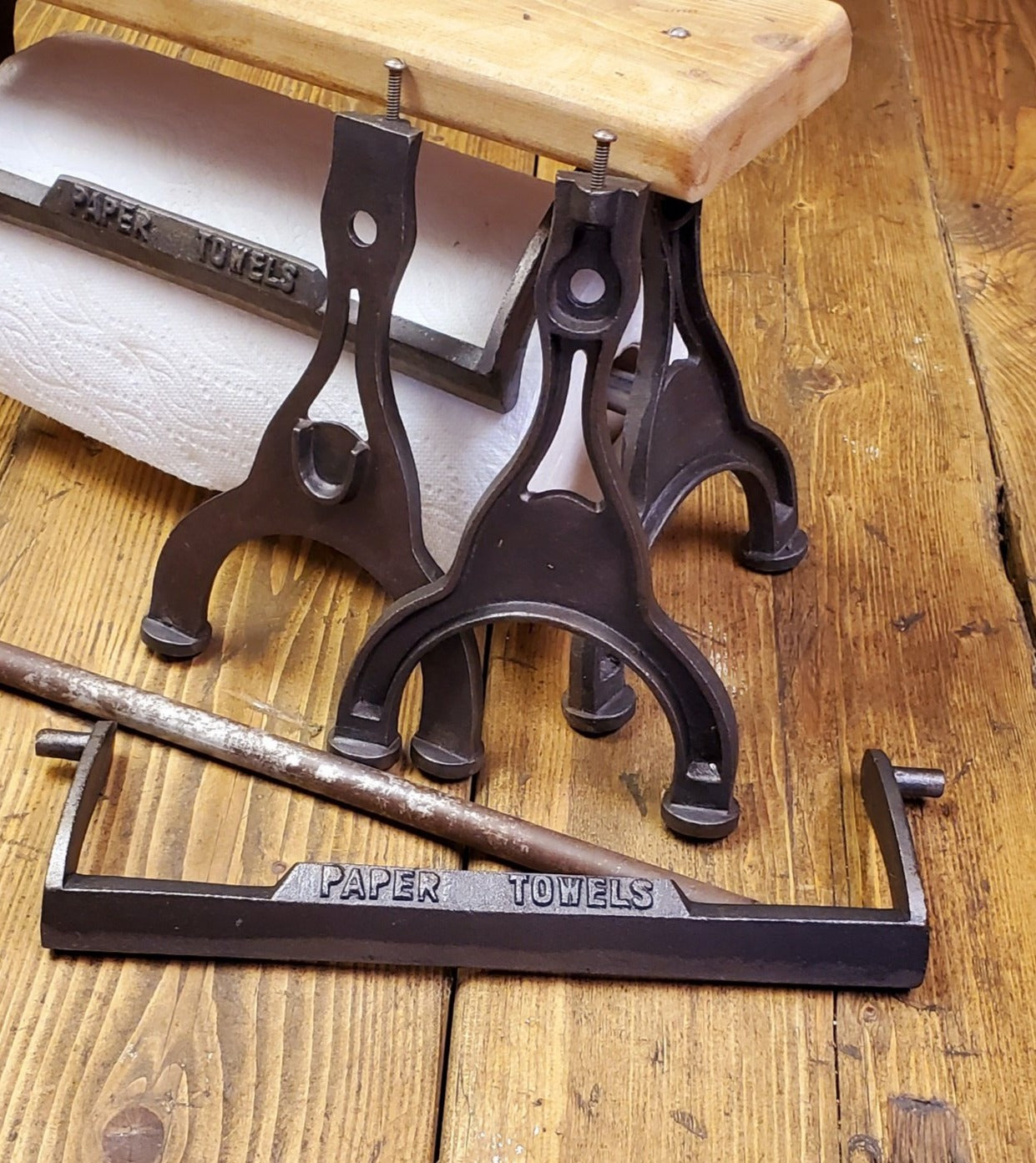In this vertically aligned rectangular image, a rustic scene is depicted. The setting features a medium brown wooden floor with vertical slats, where some wood is chipped away between two of them, revealing darker brown grains. Lying horizontally at the bottom of the image is an old-looking metal paper towel holder, with the words "PAPER TOWELS" engraved in all capital letters on the front bar. The holder, comprising a horizontal bar with vertical ends and a small knob on each end, holds a roll of paper towels.

Set against the floor, the holder also features a black, rusted diagonal bar, adding to its aged appearance. Alongside the main holder, there is a light beige rectangular piece of wood on top, appearing like a 2x4 plank, which is likely intended for assembling the holder. Additionally, the image shows brown metal legs, possibly parts of the holder, curving at the bottom with small circular feet and screws at the top, ready for attachment. The entire setup suggests an assembly process, blending the natural wood textures with the aged metal components, illustrating the rustic charm of the paper towel holder in its environment.